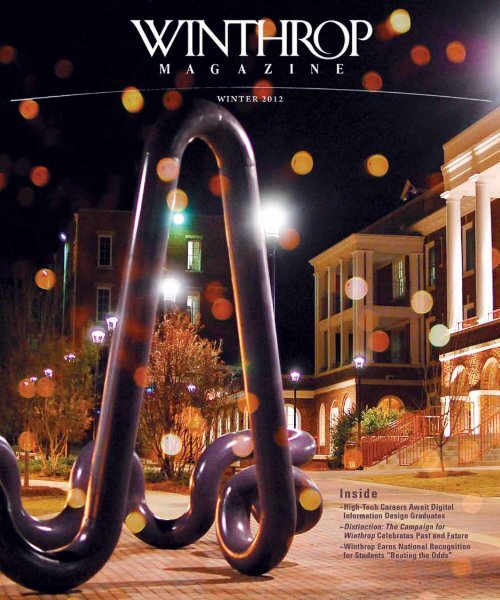The magazine cover on display is "Winthrop Magazine," from Winter 2012. The cover prominently features an outdoor night-time scene of Winthrop University's campus, with tall brick academic buildings illuminated against the dark sky. In the foreground, there's a large, intricate art sculpture resembling a looping, tubular structure that adds a dramatic focal point to the scene. The ground is lined with brick walkways, and autumnal trees with orange leaves frame the composition. The title of the magazine is emblazoned at the top in white capital letters, and beneath it, the issue's timeframe is noted. The bottom right corner of the cover includes text detailing some of the featured articles: "Inside: High Tech Careers Await Digital Information Design Graduates," "The Campaign for Winthrop Celebrates Past and Future," and "Winthrop Earns National Recognition for Students Beating the Odds." The careful play of campus lights and reflections throughout the image further enriches the visual appeal of this detailed and vibrant magazine cover.